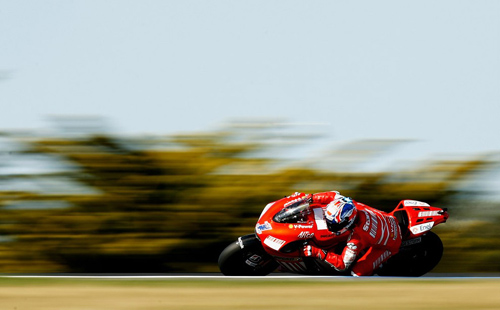In this outdoor, landscape-oriented photograph, a professional biker is captured mid-race, taking a sharp corner on a red and white race motorcycle. The rider is dressed in a red and white racing suit, complemented by a helmet adorned with blue and red accents, and both the bike and the rider's suit are emblazoned with various white logos and sponsors. The motorcycle is dramatically tilted, almost parallel to the ground, with the biker's left elbow and knee nearly touching the surface, demonstrating expert maneuvering at high speed. The background is extensively blurred due to the incredible velocity, showcasing a blend of green from trees and shrubbery, and a blue sky, while the track beneath the bike is a mix of brown and tan colors. The image vividly conveys the dynamic motion and intensity of the race, with all other elements fading away to spotlight the rider's skill and the vivid colors of his gear and motorcycle.